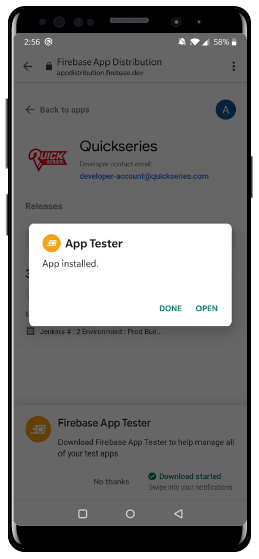The image depicts a smartphone, likely a Samsung Galaxy or similar Android device, displaying a notification that an app called "Quick Series" has been installed. The screen offers two options: "Done" and "Open." The device shows a time of 2:56 PM and a battery level of 58%. The entire phone is visible in the image, clearly indicating its make and model are not from Apple's iPhone line. The app "Quick Series" is unfamiliar to the narrator, who expresses uncertainty about its relevance. The phone's interface and details such as battery life and time offer additional context to the scenario.